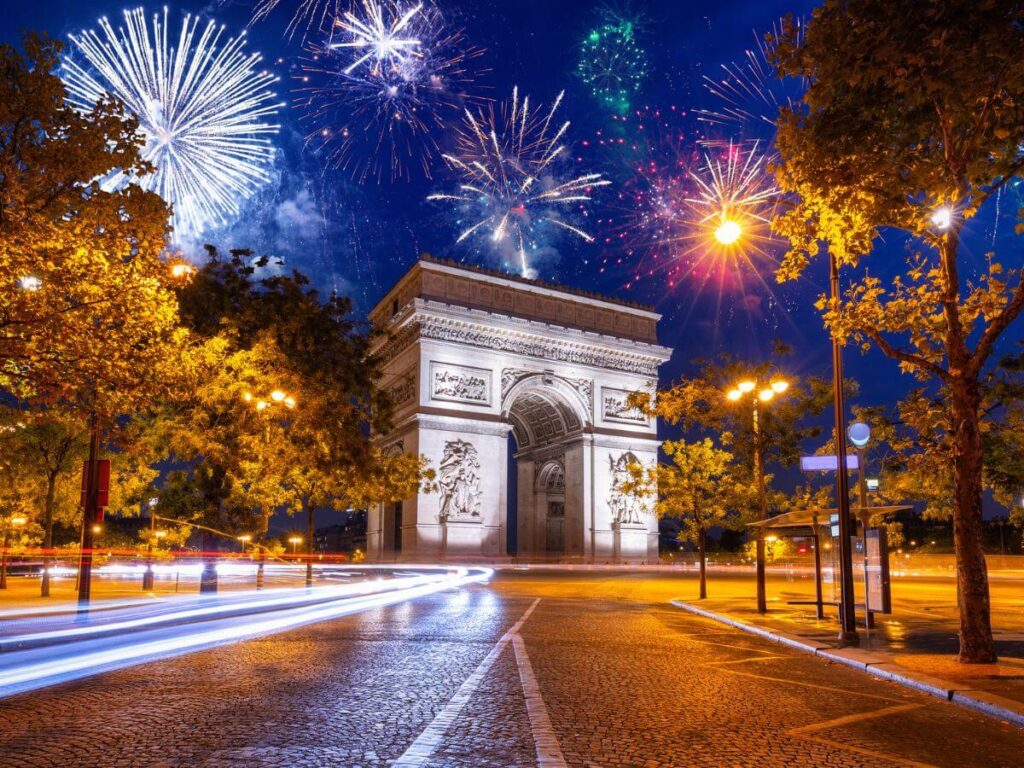The image showcases a captivating scene, possibly a photograph or a computer-generated composite, featuring a wide roadway leading up to an imposing structure composed of massive pillars forming a grand, door-like gateway. Intricate engravings and various representations adorn the surface of this monumental edifice. Above this structure, against a backdrop of a blue-tinged nighttime sky, an array of vibrant fireworks burst forth in a spectacular display. The fireworks, resembling mortar shells, explode in a multitude of colors, enhancing the festive ambiance. Framing the majestic scene, neatly planted trees punctuate both sides of the roadway, emerging from concrete planters, suggestive of a well-maintained park setting. The careful placement of the trees adds a harmonious balance to the composition, making it an evocative and meticulously crafted image.